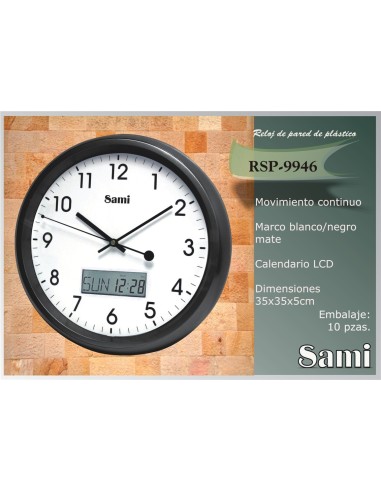The image showcases an advertisement for a multifunctional clock set against a primarily white background. At the center of the composition is a rectangular card, resembling a business card, framed by a gray border. To the left of this card, the clock is displayed over a wooden background. The clock itself is a hybrid model combining both an analog and a digital display. The analog face is complemented by a digital screen located beneath the center, which shows the date "12-28." Various shades of brown, black, white, and green adorn the clock, giving it a rustic yet modern appearance. 

To the right of the clock, there is a vertical space filled with text written in a different language, possibly Spanish. This section includes detailed features of the clock alongside the model number, RSP9946, and the brand name, Sammy. Surrounding the entire image is a gray border, enhancing its framed advertisement look. The overall layout and design suggest a professional promotional piece, likely highlighting the clock's multi-functional capabilities and aesthetic appeal.